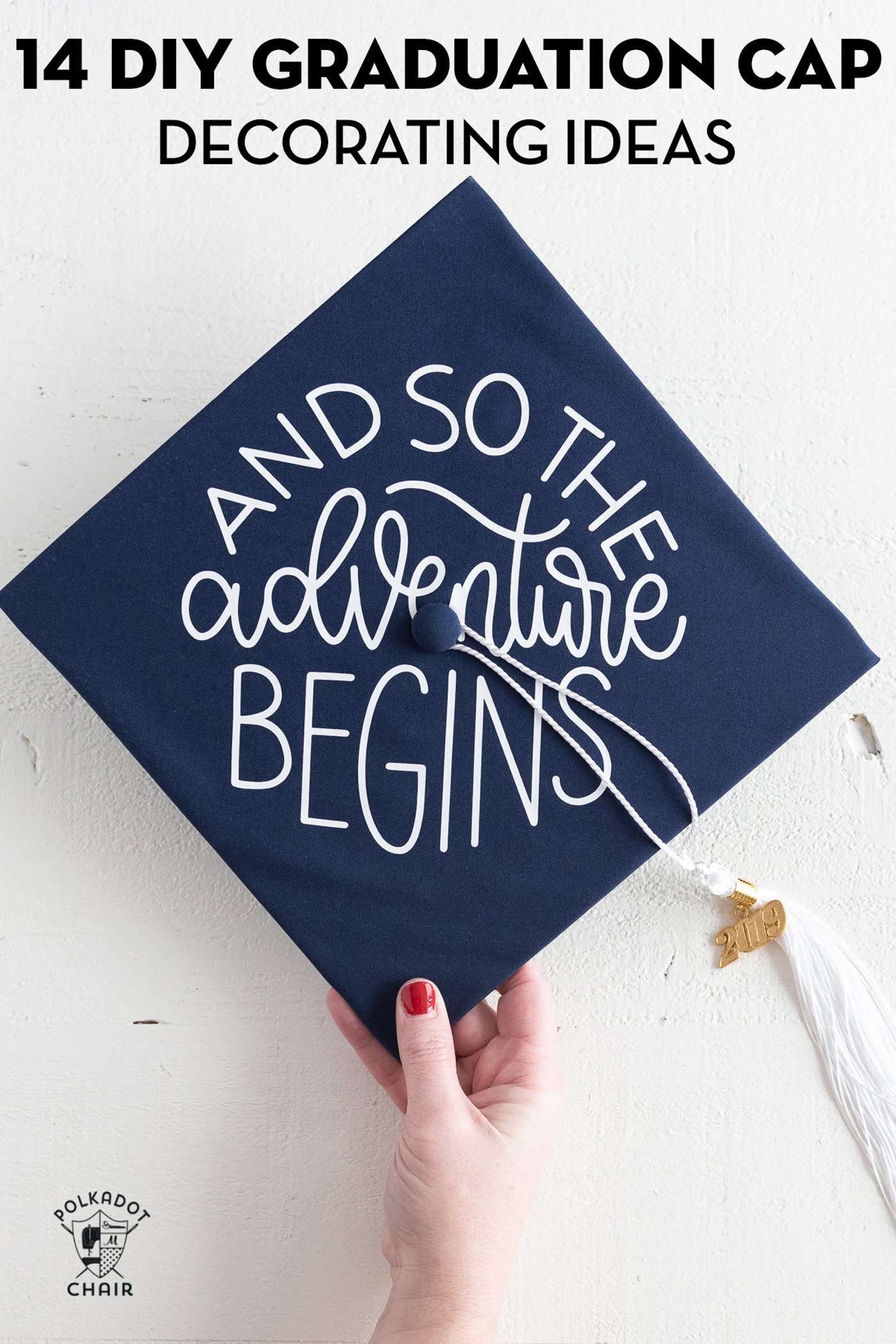The photograph features a Caucasian hand with red fingernails holding a navy blue graduation cap from the top, set against a white stucco wall. The cap is positioned so it resembles a diamond and bears the simple white text, "and so the adventure begins." A white tassel runs diagonally to the right, adorned with a golden 2019 charm. At the bottom left of the image, there's a shield emblem featuring an electric drill on the left and a letter "M" with polka dots on the right, alongside black text that reads "polka dot chair." At the top of the image, black text announces, "14 DIY graduation cap decorating ideas."